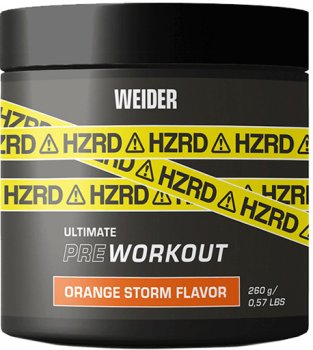The photograph showcases a cylindrical black container of pre-workout powder with a matching black lid. The front of the container prominently features the brand name "WEIDER" in bold white letters. Below the brand name are three overlapping yellow hazard stickers. Each sticker is inscribed with "HZRD" alongside a triangle containing an exclamation mark, denoting caution. Beneath the hazard warnings, the label reads "Ultimate Pre-Workout" in a striking font. An orange rectangle just below this text highlights the flavor of the supplement, stating "Orange Storm Flavor" in white letters. The container also indicates its weight, which appears to be either 250 or 260 grams (0.57 pounds), though the exact number is slightly obscured.